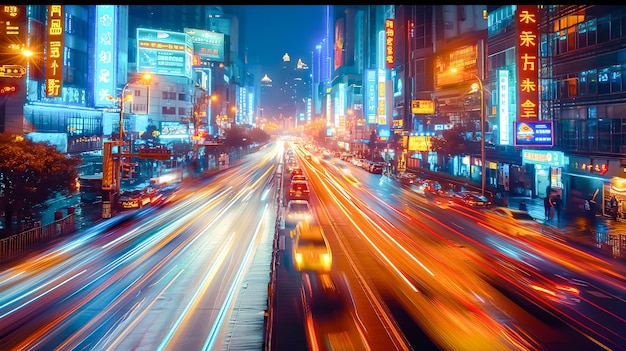The photograph showcases a bustling nighttime urban street scene from either China or Japan, captured with a time-lapse technique. Dominating the center of the three or four-lane road are colorful motion lines—yellow, red, orange, and blue—created by the high-speed movement of cars. The left side of the street is enveloped in a bluish hue while the right side glows with orange tones. Illuminated street lamps cast an orange glow, and multi-storied buildings on either side are adorned with brightly lit store signs, billboards, and advertisements in blue and orange. These signs predominantly feature Asian characters, adding to the vibrant cityscape filled with high-rises and storefronts. Despite the apparent late hour indicated by the dark blue sky, the scene remains lively with cars zipping by and only a few pedestrians visible, providing contrast to the motion-filled street. In the distant background, very tall buildings tower over the scene, enhancing the dynamic and energetic atmosphere of this urban setting.